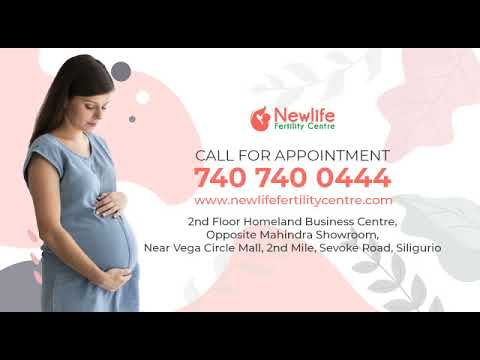The advertisement for the New Life Fertility Center features a serene and hopeful image of a pregnant woman on the left side. She has brown hair, styled down, and wears a light blue maternity dress while tenderly holding her belly, gazing downward. The center of the ad prominently displays the text "New Life Fertility Center" and "Call for appointments: 740-740-0444," both in red. Below, the website address, "www.NewLifeFertilityCenter.com," and detailed location instructions are provided, indicating the clinic is on the second floor of Homeland Business Center, opposite Mahindra showroom near Vegas Circle Mall. The background is artistically adorned with blurred red and black leaves transitioning into gray and light pink shades, with gray and white bubbles adding depth to the composition. The advertisement's layout, with the woman on the left and informative text and visuals throughout, aims to draw attention to the clinic, offering hope to individuals and couples seeking fertility solutions.